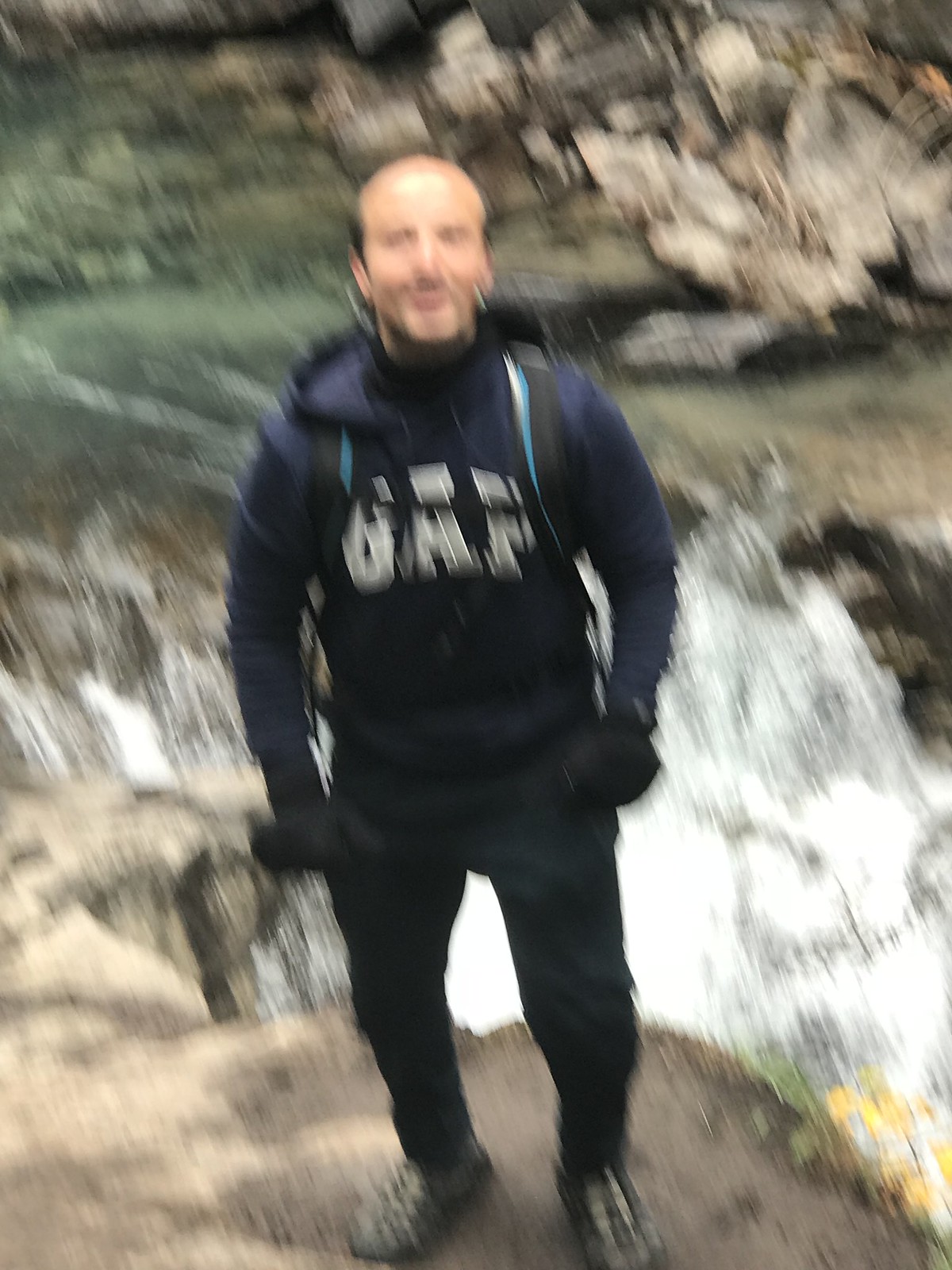The image shows a blurry snapshot of a man posing in front of a churning river and a small waterfall. He is wearing a blue GAP hoodie with white letters, dark pants, and hiking boots with visible silver grommets. He has on dark gloves and a backpack with black and blue stripes, the straps clearly visible on his chest. The man has male pattern baldness, characterized by a shiny head with dark hair above his ears, and a gray or stubbly beard. He appears to be slightly bent at the knees, possibly smiling. The river behind him, framed by large brown and grey rocks, shows water pooling in the upper left before cascading down in a frothy rush. A yellow branch is visible in the bottom right corner, adding a touch of color to the rocky, natural setting.